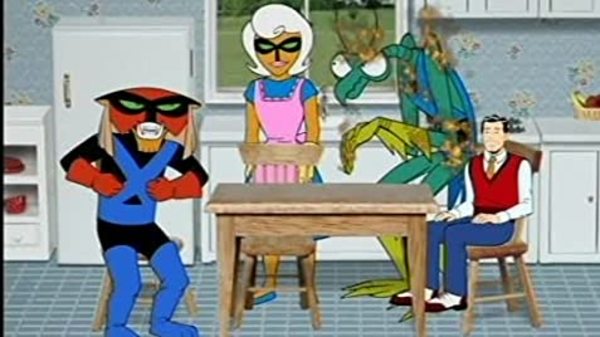In this surreal animated scene set in a vintage 1960s kitchen, various fantastical characters gather around a central wooden table. The kitchen backdrop features a boxy, vertically rectangular white refrigerator and a countertop with a sink, adorned with blue floral wallpaper and a bluish floor. At the table stands a woman with white hair, which appears to be a wig, wearing a blue dress and a pink apron. She has a black mask over her eyes, adding to the surreal atmosphere. To her right is an oversized, anthropomorphic insect resembling a praying mantis, colored blue with long green gloves, staring intently at her. Adjacent to the table is a small man seated in a wooden chair; he has dark hair and dons a red vest over a white button-down shirt, paired with blue pants and blue-and-white shoes. On the left side of the table stands a peculiar figure dressed in a blue superhero-like outfit with red rubber gloves and a wide red mask resembling a cat's face. This eclectic mix of characters brings a whimsical and uncanny feel to the otherwise nostalgic kitchen setting.